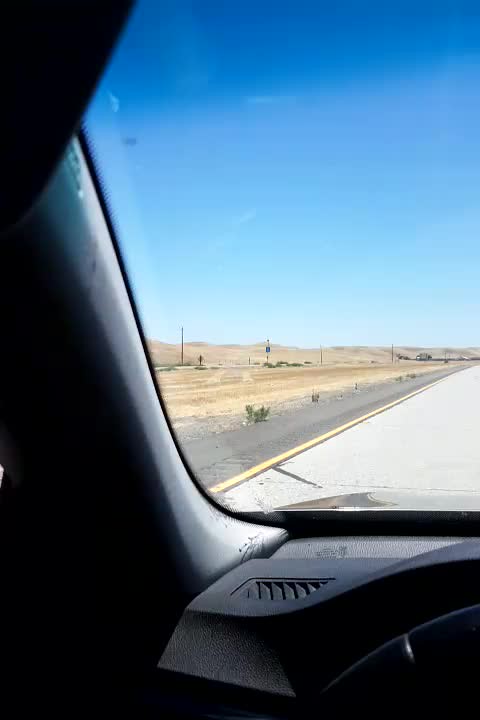The image is a vertically rectangular frame viewed from the lower left corner of a driver's side windshield, including the end of the dashboard on the right and the windshield frame extending upwards on the left side. The vehicle's interior is gray. Through the window, the left side of the car's hood is visible, leading to a white paved area that runs diagonally upwards to the right. Beyond this, there is a narrow stretch of gray paved road, with a yellow line marking the boundary between the white and gray surfaces. In the distance, barren land and a range of hills stretch across the horizon. The sky above is a clear, bright blue, adding a vivid backdrop to the scene.